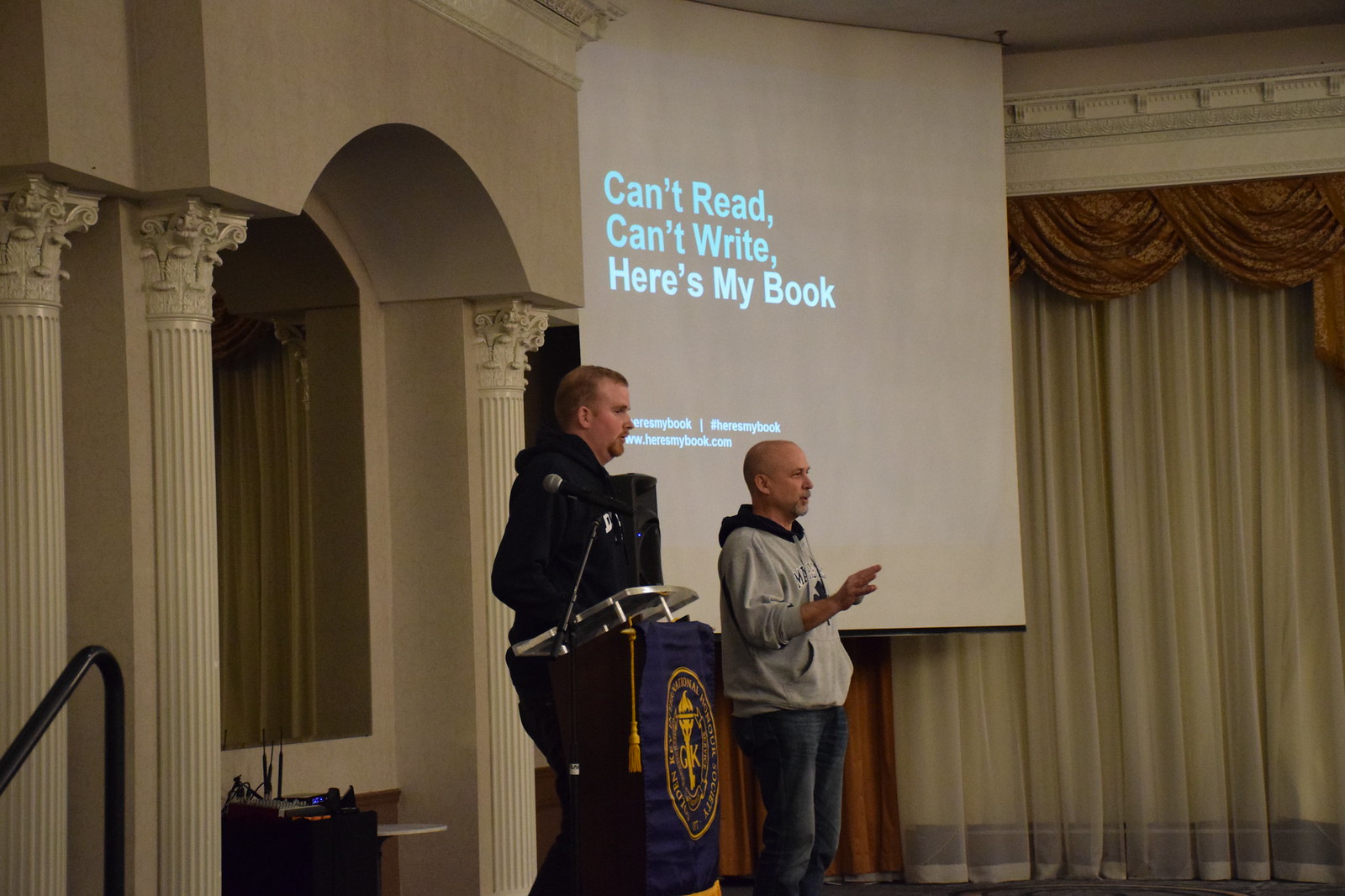In this image, a pair of middle-aged men are in the midst of giving a presentation in an ornate venue, possibly a grand ballroom. The room is richly decorated, featuring beautifully carved pillars, intricate ceiling trim, and luxurious drapes and curtains that span from floor to ceiling, accented with gold fabric swags and crown molding. 

Centered in the image is a podium, which appears to have a glass top, adorned with a blue banner displaying a yellow logo or seal and a yellow tassel. The podium is equipped with a microphone stand. Behind the podium, slightly off-center, stands a tall man with cropped hair and a short beard, dressed entirely in black. To his side, a shorter bald man with a similar beard is clad in blue jeans and a grey hoodie. He has his right hand raised as if addressing the audience.

Projected on a large screen behind them are the words, "Can't Read, Can't Write," followed by, "Here's My Book," and a web address, www.heresmybook.com. Additional sound equipment is visible behind them, along with a staircase railing on the left side of the image, suggesting the men are on a stage. Despite the clarity of their presentation setting, the audience remains unseen, providing no context for their reactions.